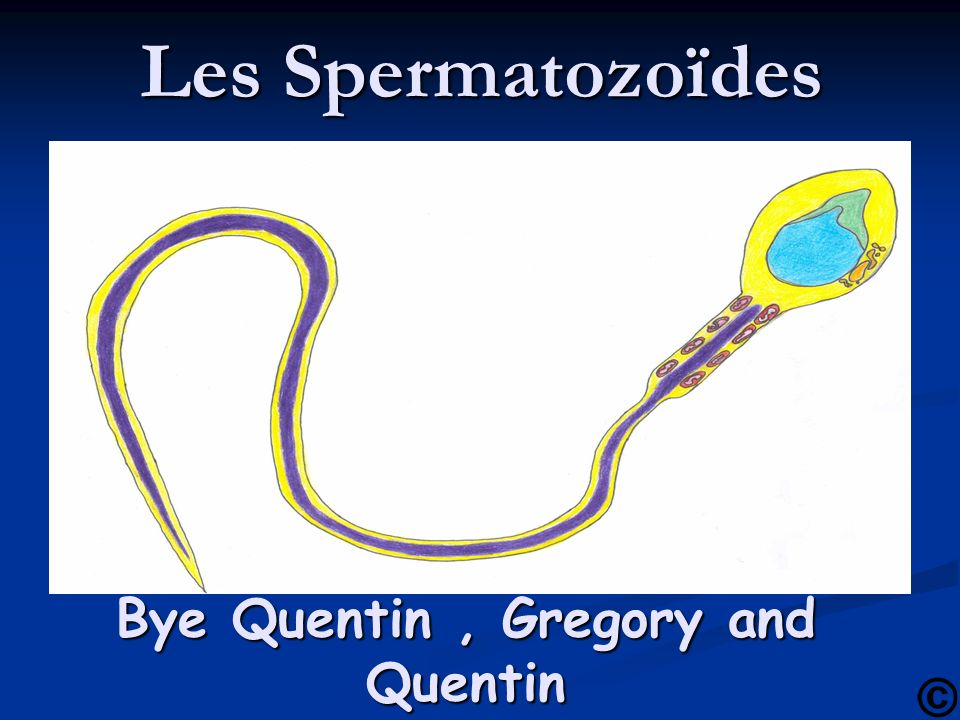The image appears to be a hand-drawn illustration of a sperm cell, depicted with a yellow head, a striped purple and yellow tail, and a blue-green main body accented with small patches of red and orange. The drawing is centered on the slide, which has a white background where the drawing is placed within a white rectangular box. The slide itself features a dark blue upper section that reads "Les Spermatozoids" in white text, suggesting a title, and a lighter blue lower section containing the text "by Quentin, Gregory, and Quentin," also in white. Additionally, the bottom right corner of the slide displays a black copyright symbol (a letter 'C' within a black circle). The slide's overall design, with its educational tone and simple layout, suggests it might be part of a PowerPoint presentation or a web page intended for educational purposes.